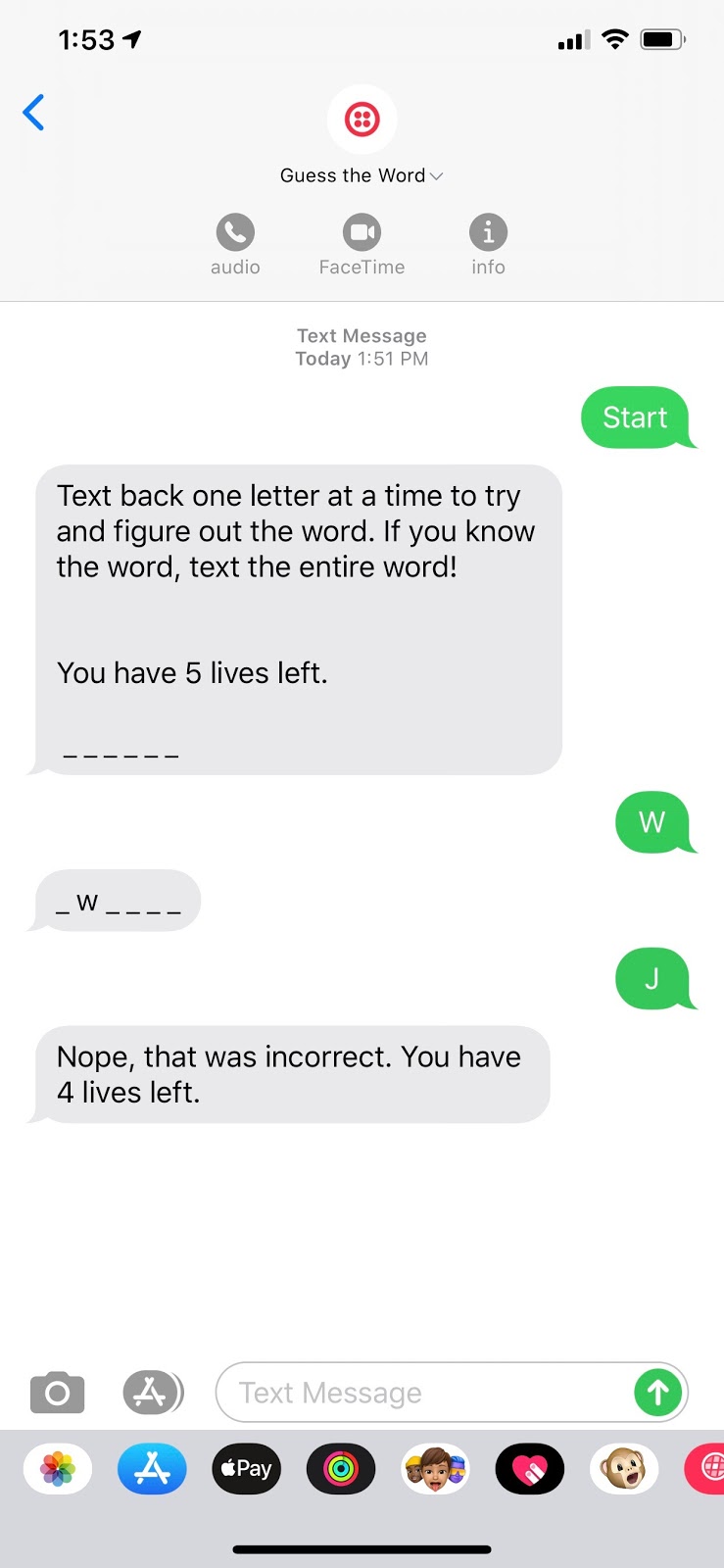This is a detailed screenshot of an iPhone operating in light mode. In the upper left corner, the time is displayed as 1:53 PM alongside a location symbol. On the upper right are icons for signal strength, Wi-Fi, and battery level.

Beneath the time, there's a blue left-pointing arrow followed by a white circle containing a red circle with four red dots inside. Below this symbol is the text "Guess the word" along with a downward arrow. Adjacent to it are icons for phone (audio), recording, FaceTime, and information.

The main body of the screen displays a series of text messages timestamped at 1:51 PM. A green text bubble on the right reads "Start." On the left, a grey bubble instructs, "Text back one letter at a time to try and figure out the word. If you know the word, text the entire word. You have five lives left." Below this, six underscores represent the letters of the word to guess.

Following this, a sequence of text bubbles showcase the guessing game: a green bubble on the right with the letter "W," and a grey bubble on the left showing the partially filled word "_ W _ _ _ _." Further down, a green bubble on the right contains the text "Ched," and a grey bubble on the left responds with "Nope, that was incorrect. You have four lives left."

At the bottom of the screen, icons for the camera, App Store, text messaging for Windows, and an up arrow within a green circle are visible. Additional symbols are also present beneath these icons.

This screenshot effectively captures a text-based word-guessing game in progress on an iPhone.